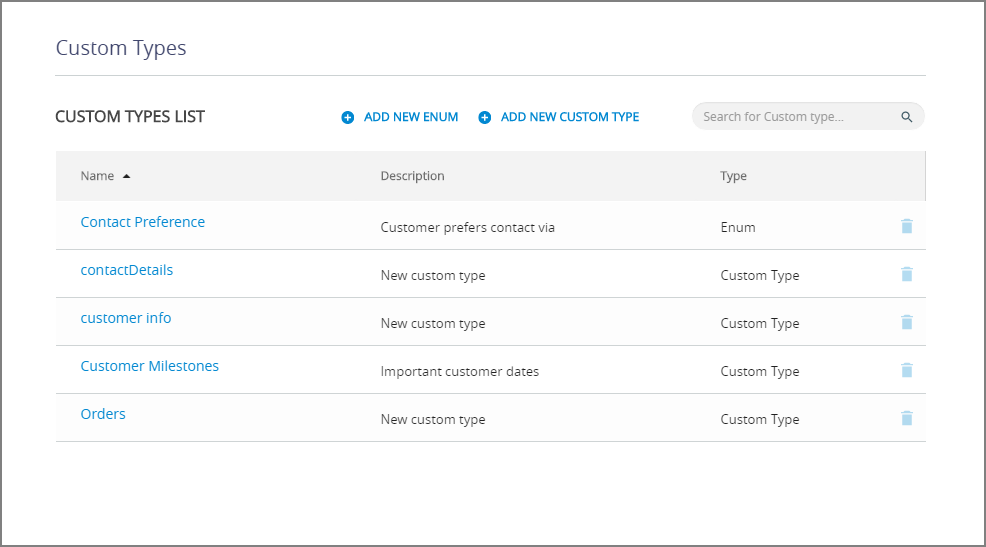A screenshot with a white background displays an interface for managing custom types. The screen prominently features lists and labels in dark gray. At the upper section, options to "Add New" and "Add New Custom Type" are highlighted, each represented by a blue circle containing a white plus sign. A search bar with the placeholder text "Search for custom type" is equipped with a blue magnifying glass icon.

Under the search bar, several columns are labeled: "Name," "Description," "Type," "Contact Preference," and "Customer," with the respective content listed beneath each heading. In the "Type" column, several entries are categorized as "enum." To the far right of each entry, blue trash can icons denote the option to delete the corresponding item.

The blue-labeled sections include:
- "Contact Preferences" under which "Customer prefers contact via" appears.
- "Contact Details."
- "Customer Info."
- "Customer Milestones" detailing important customer dates.
- "Customer Type."
- "Orders."

Each section allows for the addition of new custom types through similarly styled blue circles with white plus signs, emphasizing a user-friendly, editable interface.